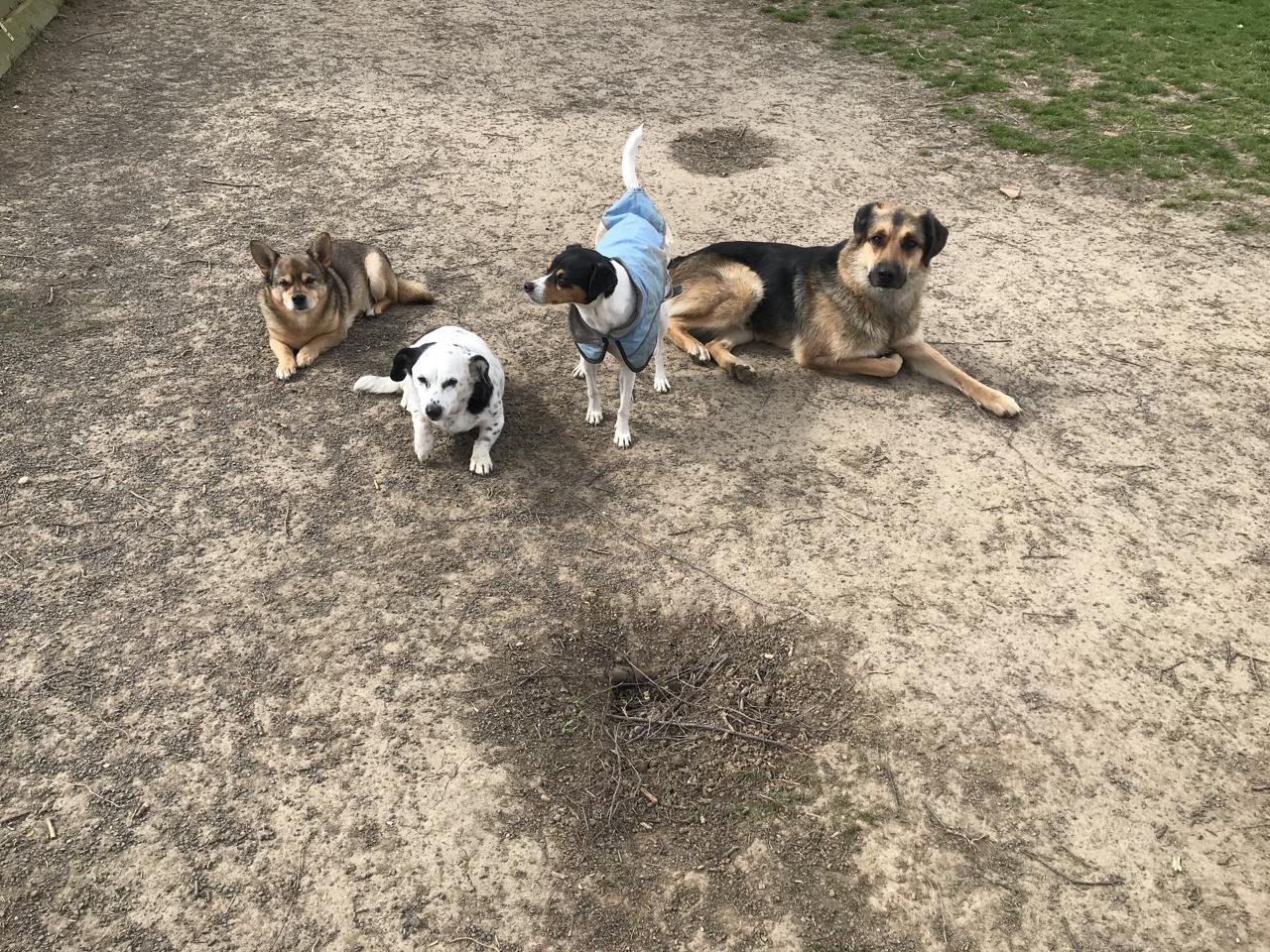This outdoor photograph captures four dogs positioned on a dirt pathway. Detailed examination reveals that three of the dogs are lying down while one stands attentively. The standing dog, a white beagle with a distinctive black head, brown face, and white muzzle, is attired in a light blue jacket and appears alert, looking away to the right.

On the far left, a small to medium-sized dog with a brown and black coat, resembling a younger pup, is lying down with its paws stretched out. Its face bears a resemblance to a wolf, with perky ears and a darker brown nose.

Next to this dog, another medium-sized, predominantly white dog with black speckles and black ears is also lying down, facing the camera.

Further to the right, the largest dog, identifiable as a German Shepherd, lies closest to the bottom right corner. This German Shepherd boasts a traditional coat pattern with tan, brown, and black colors, characterized by a black nose and ears. 

The setting appears to be a dry park area with a sparse cover of grass noticeable in the upper right of the image, partially interrupting the otherwise gravelly and twig-strewn dirt pathway. The scene suggests a calm and serene day, with the distinct absence of sunshine enhancing the focus on the contented and observant demeanor of the dogs.